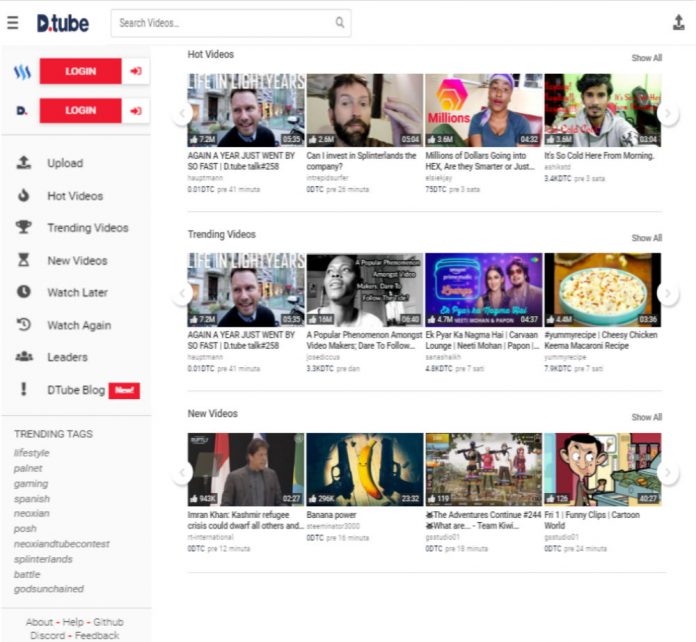The image depicts a screenshot of the DTube platform interface. In the top-left corner, the DTube logo is prominently displayed, replacing the familiar YouTube logo. Adjacent to the right, a search bar labeled "search videos" is visible. In the upper-left corner, a menu icon consisting of three horizontal lines is situated.

Below the search bar, there are two red "Login" buttons followed by two red speaker icons. Along the left-hand side of the interface, there is a vertical list of categories including "Upload," "Hot Videos," "Trending Videos," "New Videos," "Watch Later," "Watch Again," "Leaders," and "DTube Blog." Under these categories, the section titled "Trending Tags" features a vertical list of ten tags.

The main content area on the right side displays three horizontal rows of video thumbnails, each row representing different categories: "Hot Videos" at the top, "Trending Videos" in the middle, and "New Videos" at the bottom. Each row contains four video thumbnails, with the duration of each video displayed in the bottom-right corner of the thumbnail. To the right of each category title, there is a "Show All" option in gray text.

The entire interface is set against a clean white background.